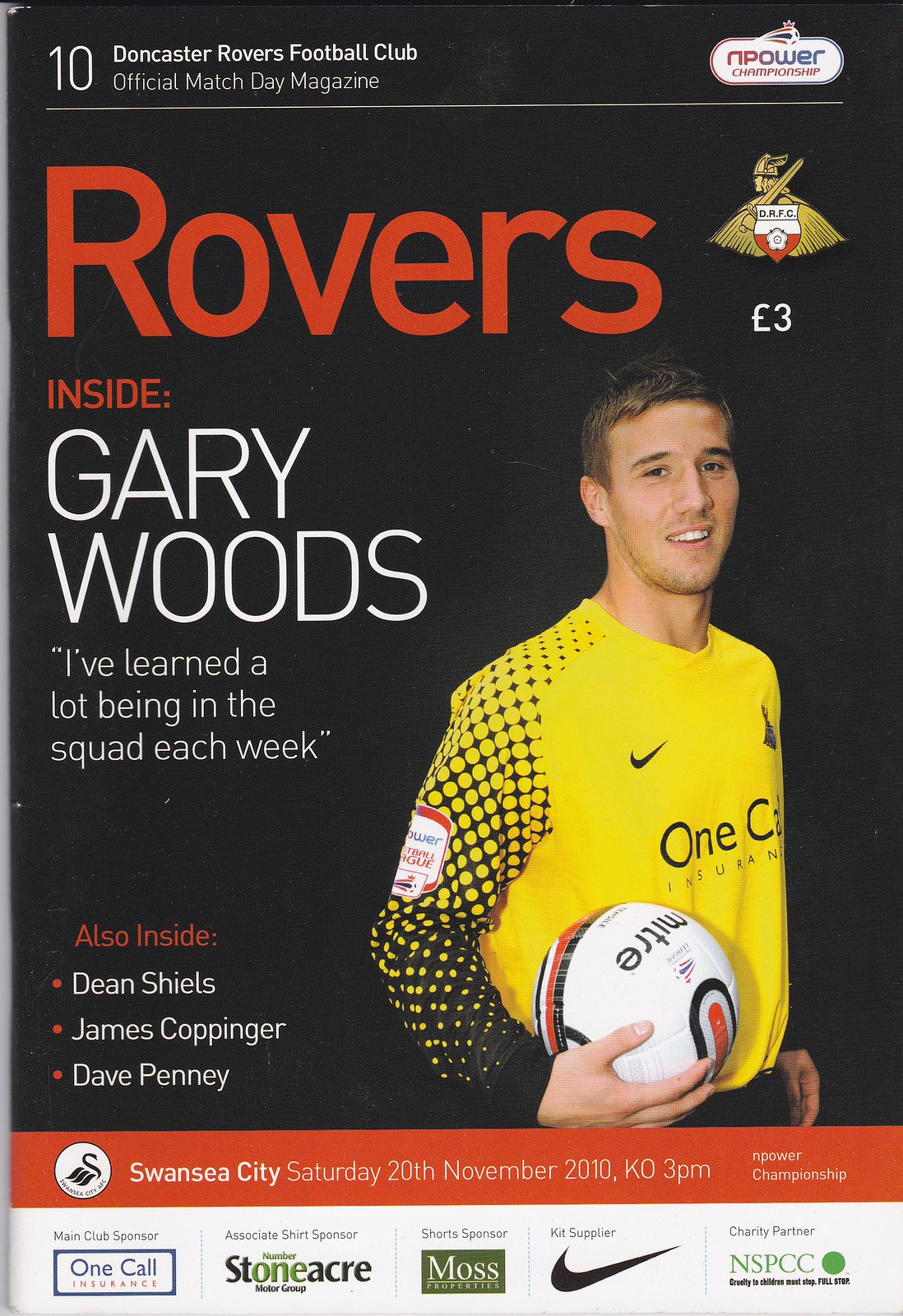This image is the cover of the Doncaster Rovers Football Club official match day magazine, issue 10. The cover features a predominantly black background with white text at the top indicating, "Doncaster Rovers Football Club, Official Match Day Magazine 10." Below this is a red line followed by "Rovers" in large red text. Underneath, in large white text, is a quote from Gary Woods: "I've learned a lot being in the squad each week." It also mentions other players: Dean Shields, James Coppinger, and Dave Penny. On the right side of the cover, there is an image of a man, likely Gary Woods, wearing a yellow long-sleeve cotton shirt partially displaying the text "One Call Insurance" due to his body's angled position. He is holding a white, black, and red striped soccer ball. 

At the bottom of the cover, it reads "Swansea City, Saturday 20th November 2010, KO 3 p.m." Additional logos and mentions of sponsors are included: One Call Insurance, Stoneacre Motor Group, Moss Properties, Nike, and charity partner NSPCC, all indicating their association with the club's kit and event sponsorship. The club's mascot, resembling a Viking with a sword, is also featured, with a shield bearing "DRFC" at the top.